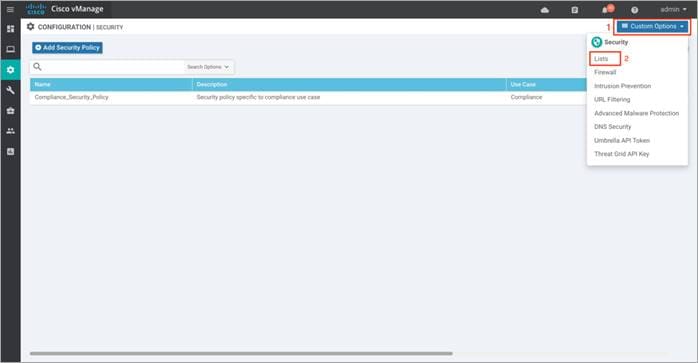This image is a blurry screenshot of a Cisco Networks webpage, specifically related to Cisco Vonage. In the upper left corner, the name "Cisco" is prominently displayed, with a three-line menu button situated to its left. Moving to the top right of the screen, several icons are visible: a cloud button, a notifications bell with an unread count (the exact number is indiscernible due to the blurriness), a help button depicted as a question mark, and an admin drop-down menu.

On the left side of the image, there's a vertical menu featuring various icons representing different sections: a settings gear, a computer screen or laptop, another settings gear, a wrench, a gift, and two people figures. The last icon at the bottom is unclear due to the blurriness.

The main content area, spanning from left to right, includes headers such as "Configuration" and "Security." Below is a drop-down menu listing various security options: "Security," "Lists," "Firewall," "Intrusion Prevention" (appearing twice), "URL Filtering," "Advanced Malware Protection," "DNS Security," "Umbrella API Token," and "Threat API Key."

Additionally, on the left side, there's a search box with partially blurred text and a down arrow indicating another drop-down menu.